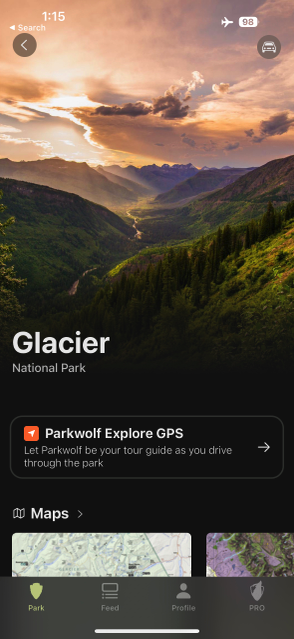The image is a screen capture taken from a smartphone that is on airplane mode, indicated by the small airplane icon in the top right corner. The time displayed is 1:15, and the battery is at 98%. The background of the website shown on the phone features a stunning mountain landscape from Glacier National Park. The scene is during sunset, with sunbeams streaming through dispersed clouds, casting a light amber hue across the sky. In the distance, the mountains appear rocky and rugged, while the nearer mountains are lush with greenery, trees, and grass. The website headline reads "Park Wolf Explore GPS," inviting users to let Park Wolf be their tour guide as they drive through the park. An arrow prompts users to click for more information, and below that, there is a map section showing two partially visible maps. The exact details of the maps are obscured, but they suggest navigation and exploration options within the national park.